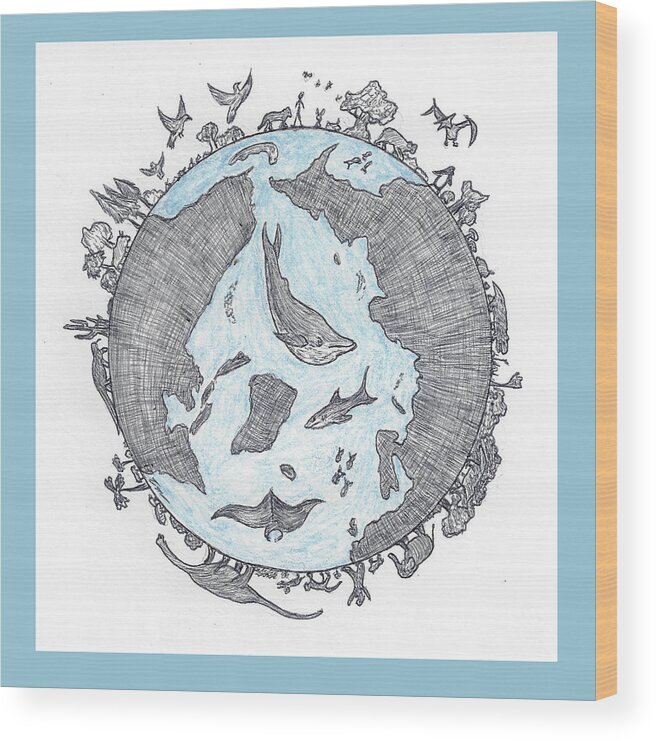This detailed, framed illustration features a whimsical, color pencil drawing of an oval-shaped globe, bordered in blue with a golden trim and mounted against a white wall. The globe itself presents an imaginative interpretation of the earth, with non-conventional landmasses depicted in gray and blue. The blue ocean teems with marine life, including dolphins, sharks, whales, manta rays, and various fish. Encircling the globe, a plethora of animals and elements from diverse ecological niches can be observed: stick figures, cacti, dinosaurs such as brontosaurus and pterodactyl, a lizard, elephants, a rabbit, a wolf, palm trees, numerous birds, and even a flying dinosaur. This fanciful artwork, almost childlike in its execution, brings together a wide array of terrestrial and avian creatures in a single vibrant tableau, exuding both creativity and a sense of global unity through nature.